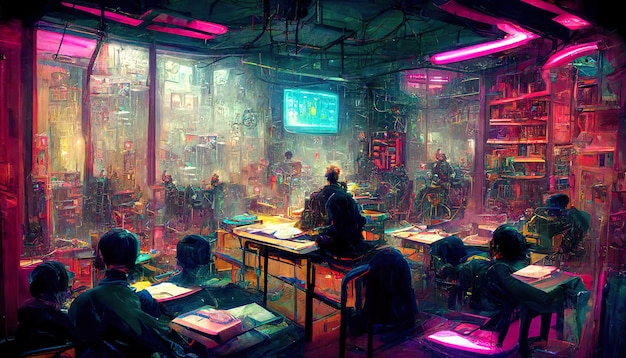The image is a vibrant and intricately detailed artwork reminiscent of both a comic book and a computer game, drenched in electric neon hues of pink and red. The scene appears to take place in a dimly lit, classroom-like setting or possibly a dingy bar, where the dominant features include large, perimeter-tracing neon lights on the ceiling that evoke the aesthetic of Tokyo's vivid nightlife, reminiscent of films like "John Wick," "Ghost in the Shell," and "Blade Runner." 

Central to the image is a large TV screen mounted on the wall, capturing the undivided attention of numerous individuals seated at desks. Each person wears bulky, dark over-the-ear headphones and is dressed uniformly in dark attire; they are depicted from behind, giving off an air of collective focus or contemplation. The room also features a well-stocked bookshelf on one side, adding a touch of intellectual ambiance. The overall composition masterfully blends bright neon lighting with a shadowy interior, making for a striking and immersive visual experience.